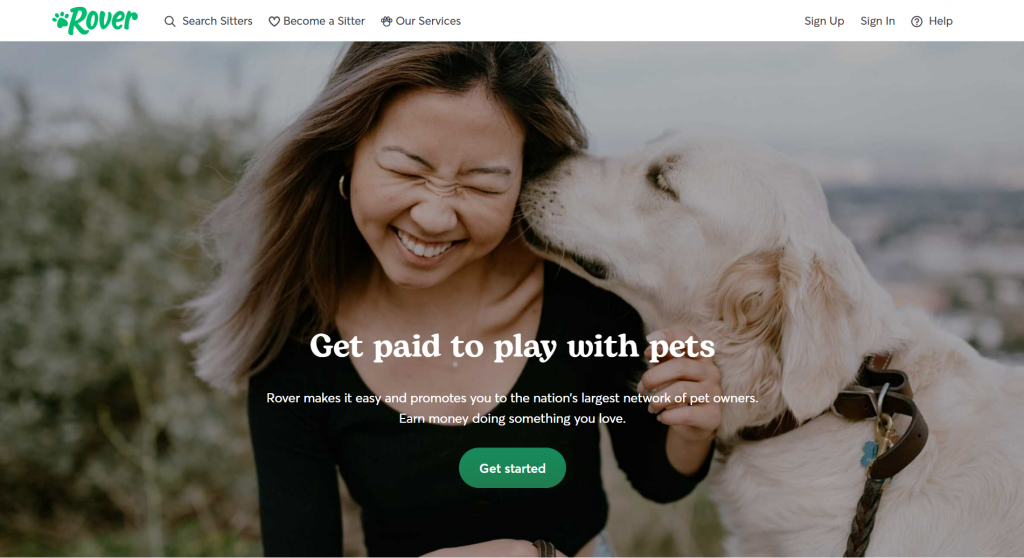This image, featured on the Rover website, is heartwarming and vibrant. At its center, a young woman of Asian descent, with long brown hair, is laughing joyfully. She has a scrunched-up nose and a radiant smile as a large, beautiful white dog affectionately kisses her left cheek. The dog's nose is nestled near her left ear, and it wears a leather collar with various tags, one appearing to be a blue bone-shaped tag. The woman, slim with visible collarbones, wears an earring on her right ear.

Above the image, the word "Rover" appears in green, accompanied by their signature paw print. The website interface includes a search bar for finding sitters, options to become a sitter, explore services, sign up, sign in, or get help. A prominent tagline reads, "Get paid to play with pets. Rover makes it easy and promotes you to the nation's largest network of pet owners." It invites users to "Earn money doing something you love," with a noticeable green oval button marked "Get Started" in white, ready to click.